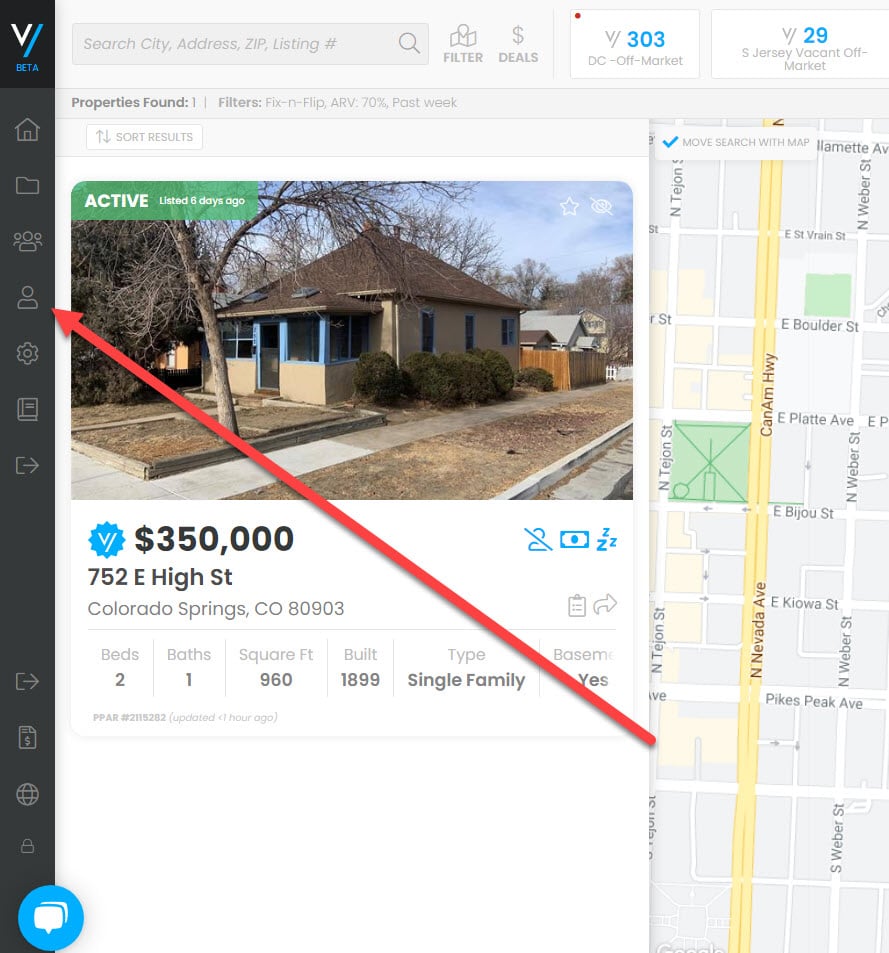This portrait-oriented image showcases a search website with a detailed interface. The website features a prominent black banner along the right side. At the top left corner, there is a distinctive logo: a white "V" against a blue slash, accompanied by the word "beta." Beneath the logo, a gray vertical bar displays various icons including: Home, Files, People, Individual Person, Settings, Book, and Return.

A striking red arrow is positioned, starting from the bottom right and pointing directly at the Individual Person icon. To the left of this bar, a rectangular information box indicates "Active Listed Six Days Ago," featuring details of a property—a small, brown house listed at $350,000, located in Colorado Springs, Colorado. The listing further details include the zip code, 2 bedrooms, 1 bathroom, 960 square feet, built either in 1980 or 1899, single-family with a basement.

The photo also includes a map displaying several streets such as Boulder and Platte Ave, and a highlighted yellow highway. At the top of the image, there are additional listings, labeled "Off Market" with the indication of 303 properties, and another "S Jersey Vacant Off Market" displaying 29 properties.

Central to the interface is a search bar reading "Search City Address and Listing," flanked by filter and deal options. Below this, there's an indicator showing the number of found properties and a white box with gray font to sort the results.